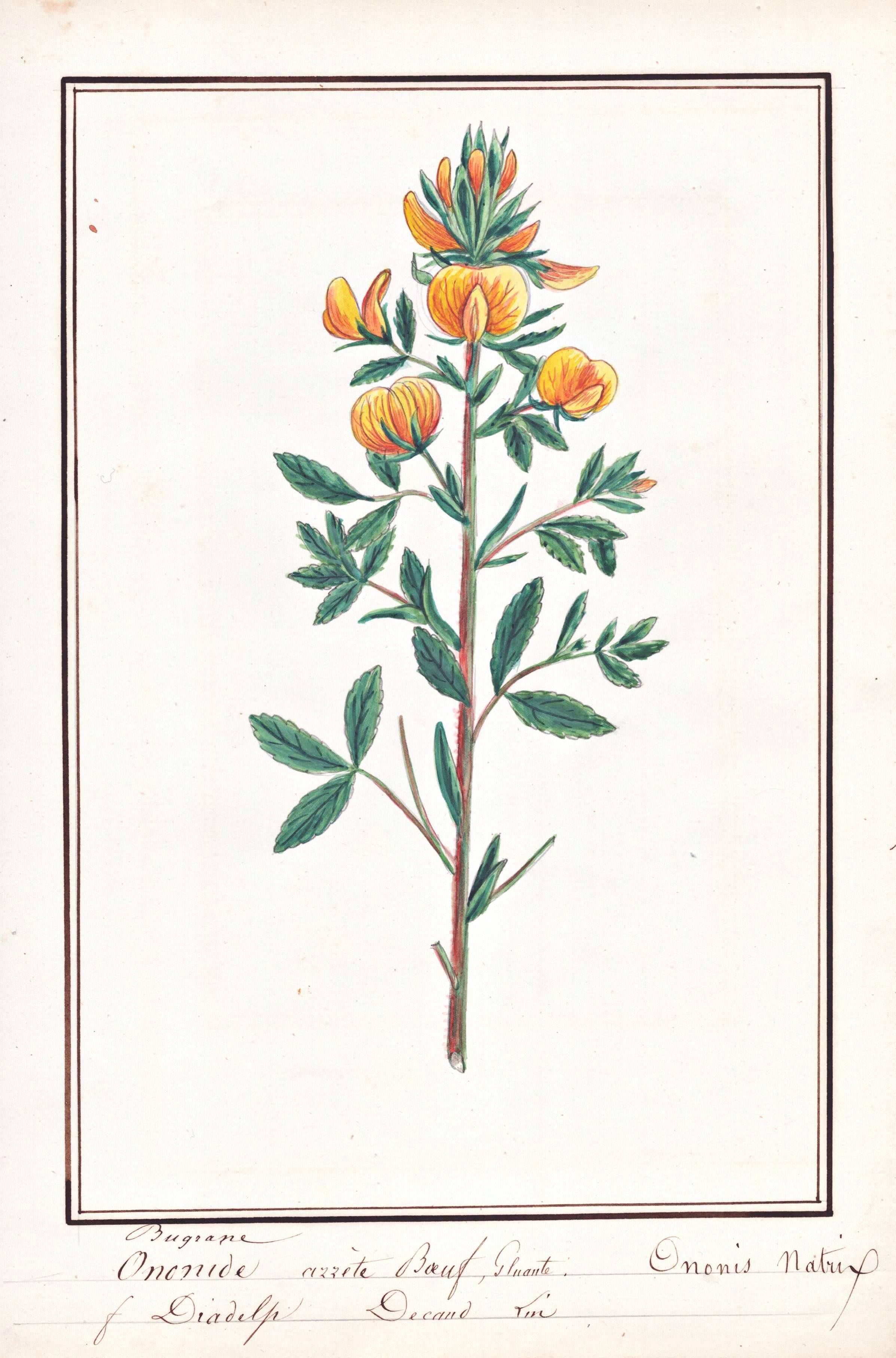The image depicts an antique styled card in portrait mode, featuring a detailed painting of a vertically positioned flowering plant. The plant, outlined with two black borders—one thinner than the other—and a light brown border, is set against a cream-colored background. It has a long, thin brown stem from which multiple smaller stems with dark green leaves extend. At the top, the plant is adorned with several tomato-shaped orange flowers, one of which is open, displaying two visible petals. The top cluster of petals resembles a Christmas tree shape intermingled with green leaves. There are some red marks towards the top left of the image, enhancing its vintage appearance. At the bottom of the card, written in light brown cursive on the white sheet of paper, are the words: "Bagrain, Onanide, Azette, Bout, Clonte, Anonis, Natree, I, Diadel, Decand, Tin."